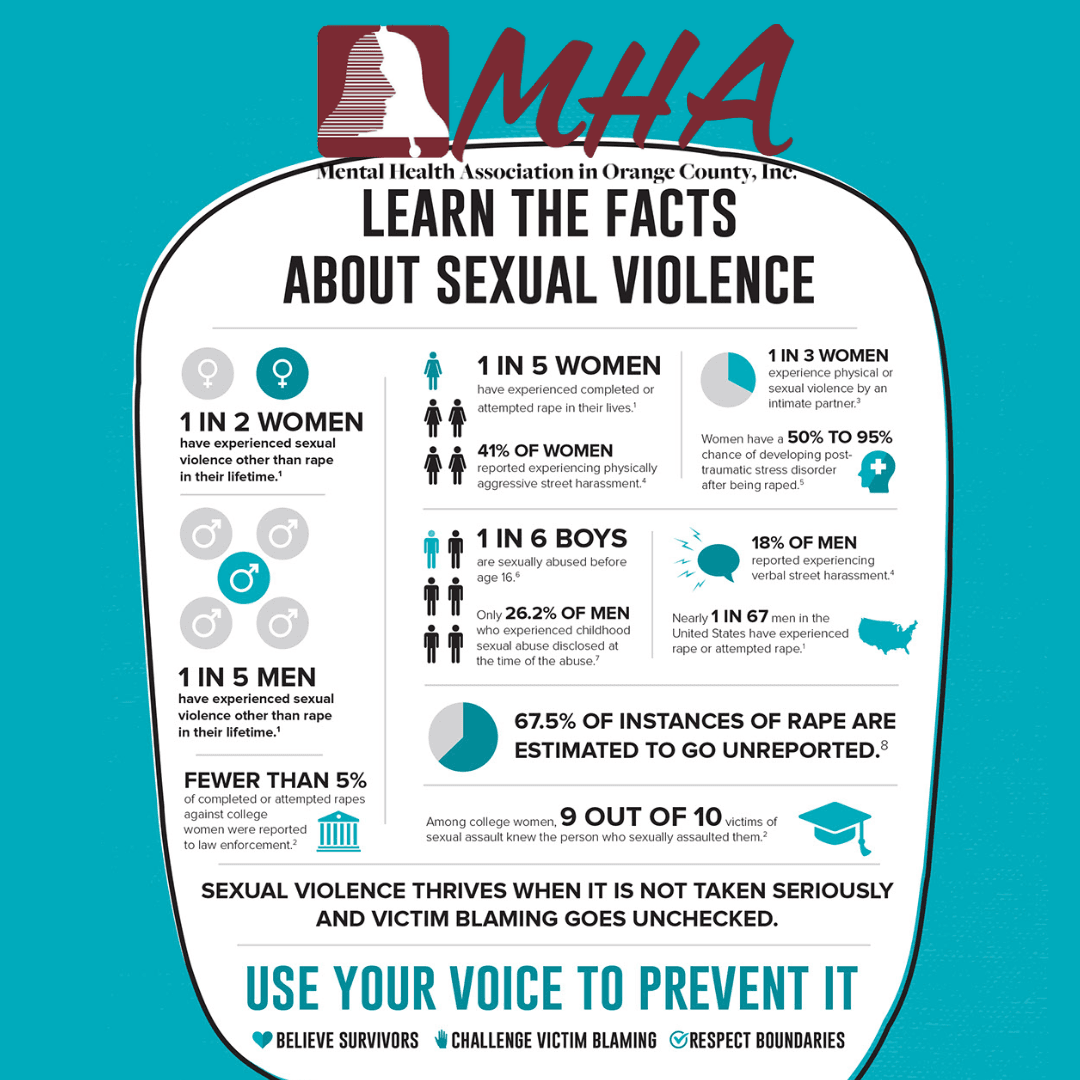This poster for the Mental Health Association in Orange County, Inc. (MHA) features a turquoise blue background with a prominent white speech bubble outlined in black. At the top, a black square contains a white and brown bell, symbolizing MHA, with "MHA" written in brown to its right. Inside the speech bubble, the organization's name—Mental Health Association in Orange County, Incorporated—is displayed in black text on a white background.

The main header, in larger black letters, urges viewers to "Learn the facts about sexual violence." Below, various statistics are presented in black text detailing the prevalence and impact of sexual violence: 
- One in two women have experienced sexual violence other than rape in their lifetime.
- One in five men have experienced sexual violence other than rape in their lifetime.
- 67.5% of rape instances go unreported.

Additional important statistics include that fewer than 5% of completed or attempted rapes against college women were reported to law enforcement, and 41% of women have reported physically aggressive street harassment. One in three women experience physical or sexual violence by an intimate partner, and there is a significant risk of developing PTSD after being raped, ranging between 50-95% for women. Among college women, 9 out of 10 victims of sexual assault knew their assailant.

The poster also features turquoise icons with key messages:
- A heart with "Believe survivors"
- A raised hand with "Challenge victim blaming"
- A check mark with "Respect boundaries"

A critical message underscores the information: "Sexual violence thrives when it is not taken seriously and victim blaming goes unchecked." At the bottom, in turquoise text, it reiterates the call to action: "Use your voice to prevent it."